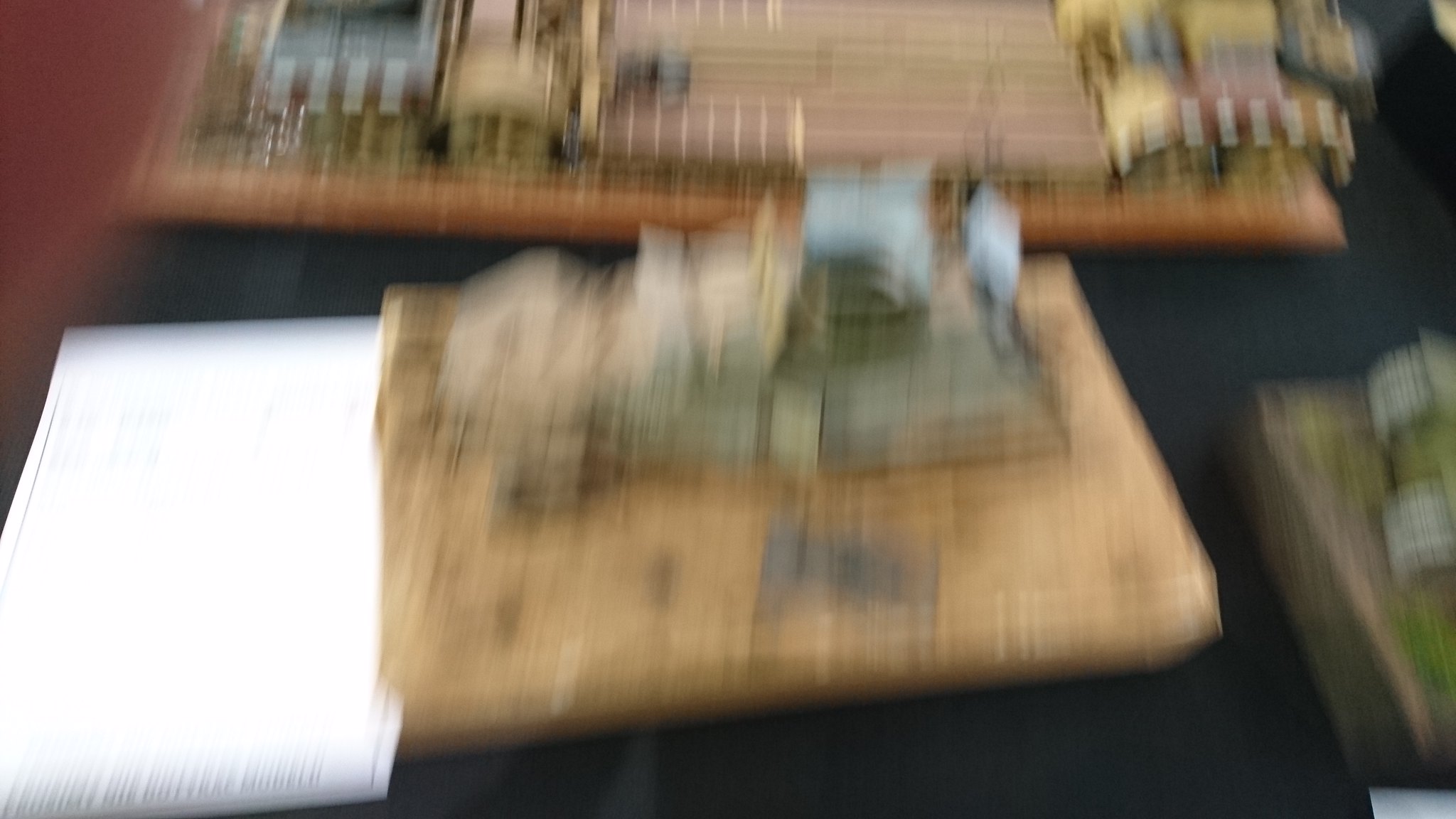The image is rather blurry, depicting what seems to be a miniature display or concept art. On the very left-hand side, a piece of white paper is visible with text at the bottom that is illegible. To the right of the paper, there is a platform supporting a detailed display. 

On the far right, elements in gray and green hues can be seen, bordered by brown edges. The background features buildings with red rooftops, and further to the left, some buildings with brown rooftops are visible. On the extreme left side of the image, there are buildings with reflective glass surfaces. An archway is also present, painted in red and white stripes, possibly part of a bridge. The scene is framed at the top and back by brown edges, adding depth to the miniature display.